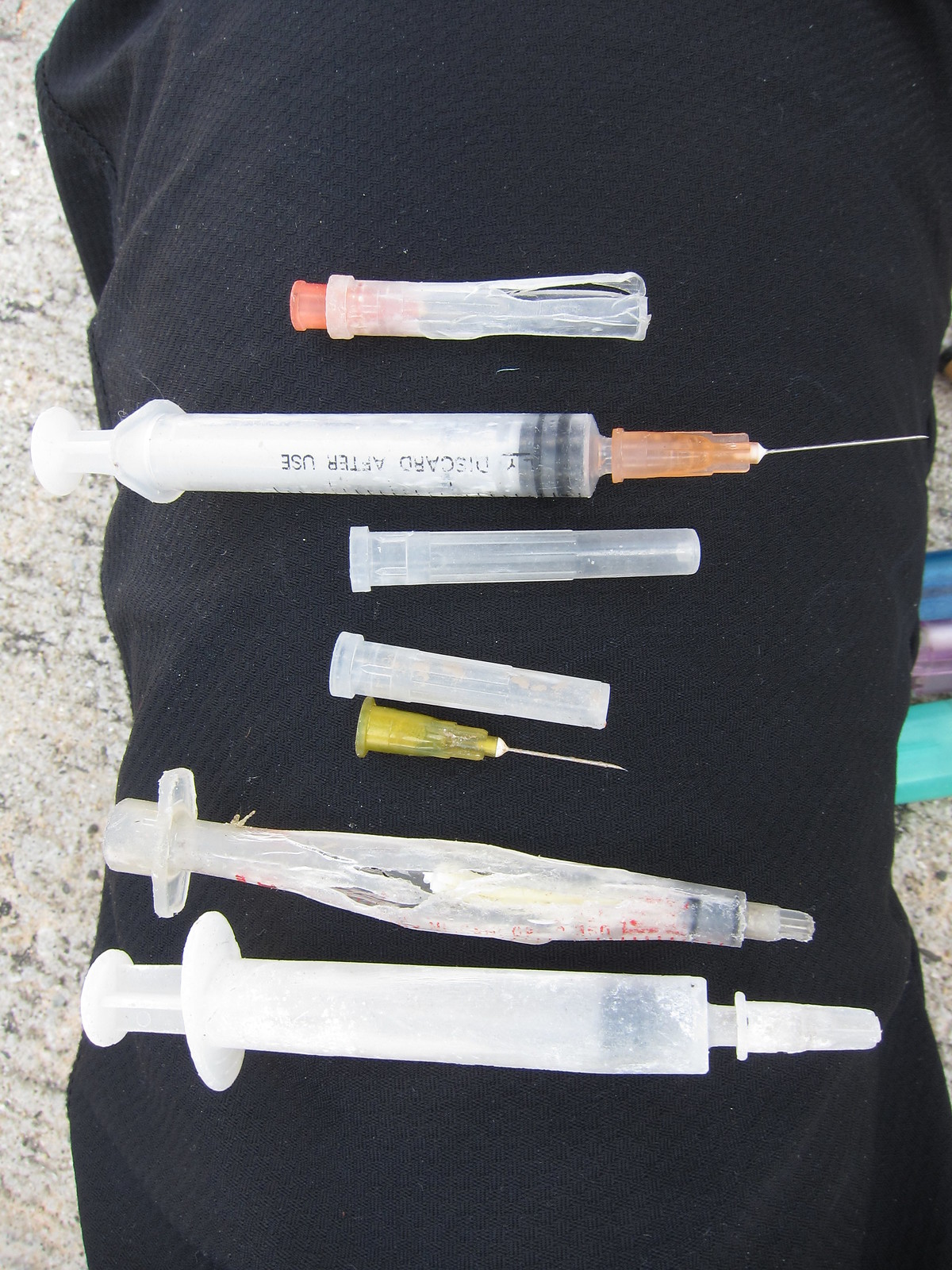The photograph depicts a tall, narrow image featuring a black piece of fabric running vertically from the bottom to the top. Flanking this strip of black fabric is a cork-like material with grey highlights and minimal quantities are visible at the sides. Several syringes, needles, and caps are strewn across the black fabric. The background beyond the fabric showcases a mixed color palette of beige, black, and soft orange.

From the bottom upwards, the first item is a larger, slightly dirty syringe without a needle. Above it lies a heavily damaged and crushed syringe, also missing its needle. Next is a yellow needle, approximately half an inch long, not attached to any syringe. Above this needle is a short, slightly dirty empty cap, followed by a second, slightly longer empty cap. Proceeding upwards, a worn-out syringe with some red markings is seen, it has no needle and appears well chewed with several holes. Next is a syringe with "discard after use" written in black, featuring an orange needle about an inch long. At the top of the arrangement is another needle with an orange base, covered by a damaged cap. All items are horizontally oriented relative to the photo.

Some of the needles are either fully exposed or capped, while others seem broken, bent, or unusable, likely picked up off the street.